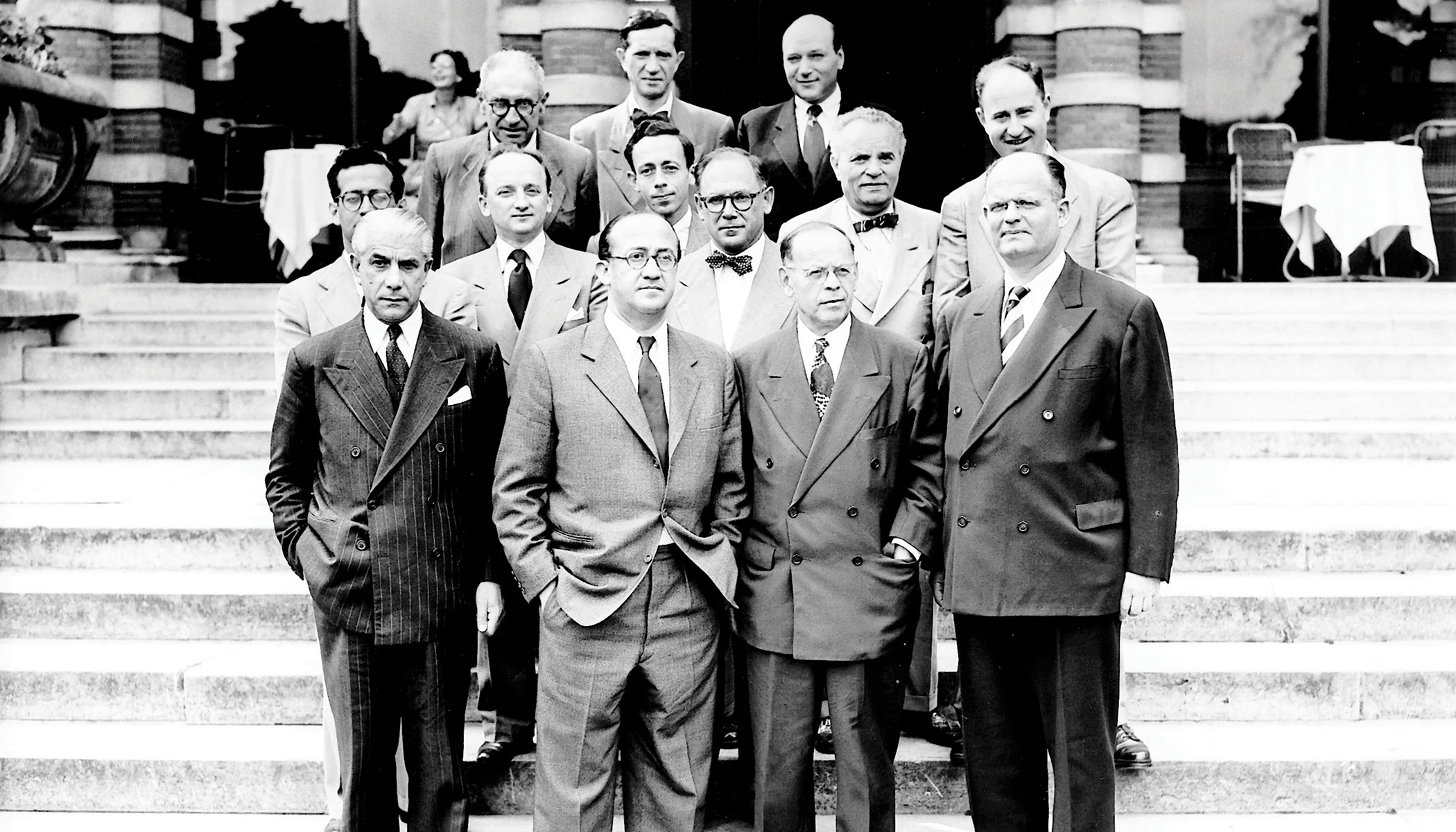This is an old black-and-white photograph, likely from the 1940s or early 1950s, showcasing a group of 13 well-dressed, light-skinned gentlemen standing on the steps of a building. The men are all wearing business suits, some with standard long ties and others with bow ties. A few of the gentlemen have glasses, and their expressions range from happy to neutral to unhappy. Some of them have their hands in their pockets, except for a man in a black pinstripe suit who has his left hand out. 

In the background, the staircase dominates the scene, leading up to a landing with a table covered in a white tablecloth and surrounded by chairs. On the left side at the top of the staircase, a woman is seated at another table. The image appears to capture a significant moment or accomplishment, as the gentlemen are grouped together for what seems to be a formal photograph commemorating an important project.